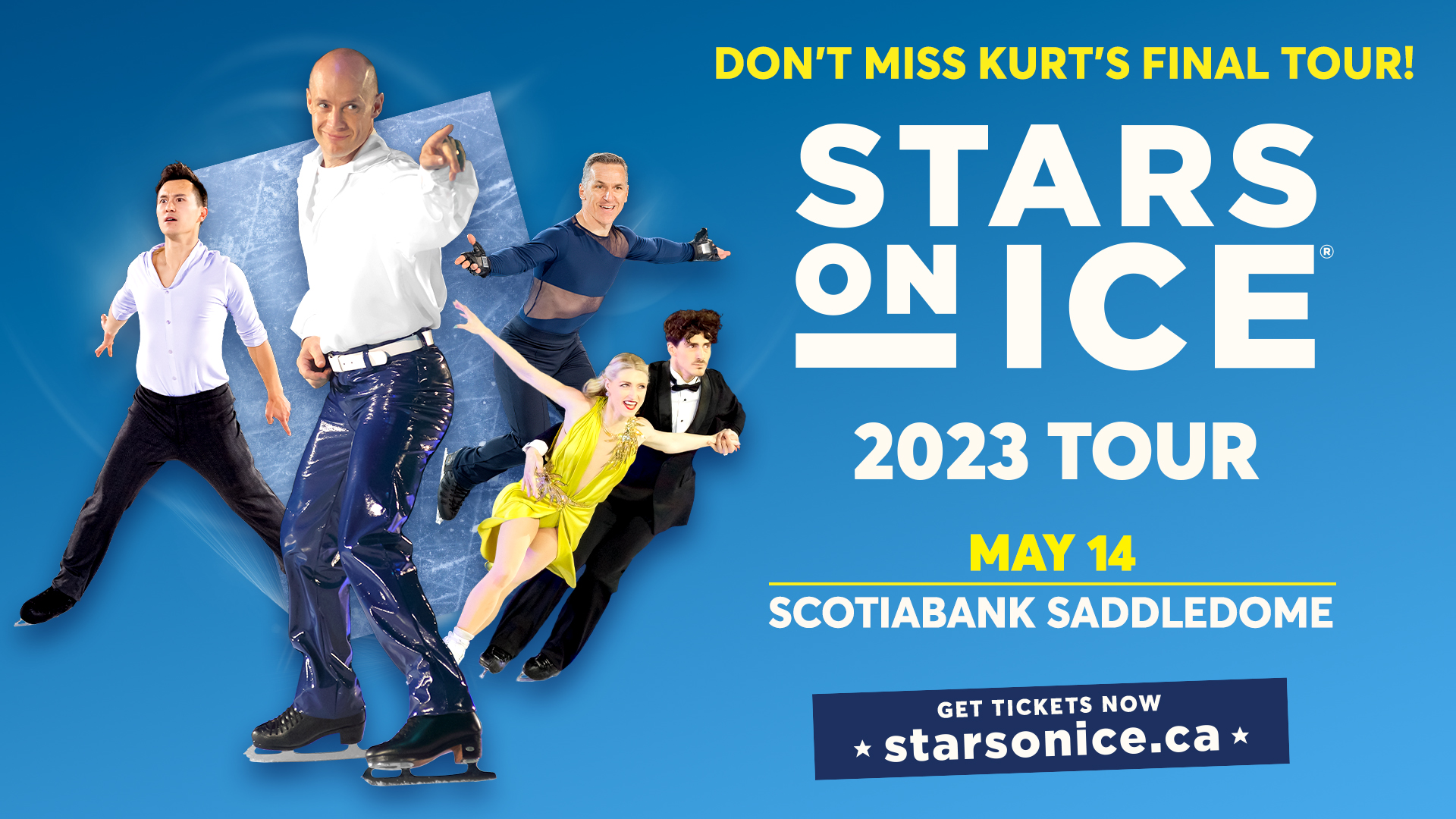The poster for Stars on Ice 2023 Tour, featuring Ms. Kurt's final tour on May 14 at the Scotiabank Saddledome, is a vivid blue with eye-catching yellow and white text urging viewers to get tickets at starsonice.ca. The montage showcases various skaters on the ice, both casually and formally dressed, against the dynamic blue backdrop. Prominently in the foreground, a smiling man in jeans and a white shirt points outward, engaging the audience. To his side, another skater in black jeans and a white shirt glides with legs wide apart. In the background, a man in black pants and a blue shirt executes an impressive jump. Capturing attention towards the viewer is a formally dressed couple; the woman, elegant in a short yellow dress, skates with her arms extended, accompanied by a man in a tuxedo who gently holds her waist. This ensemble of skaters creates a visually compelling invitation to the celebratory event.